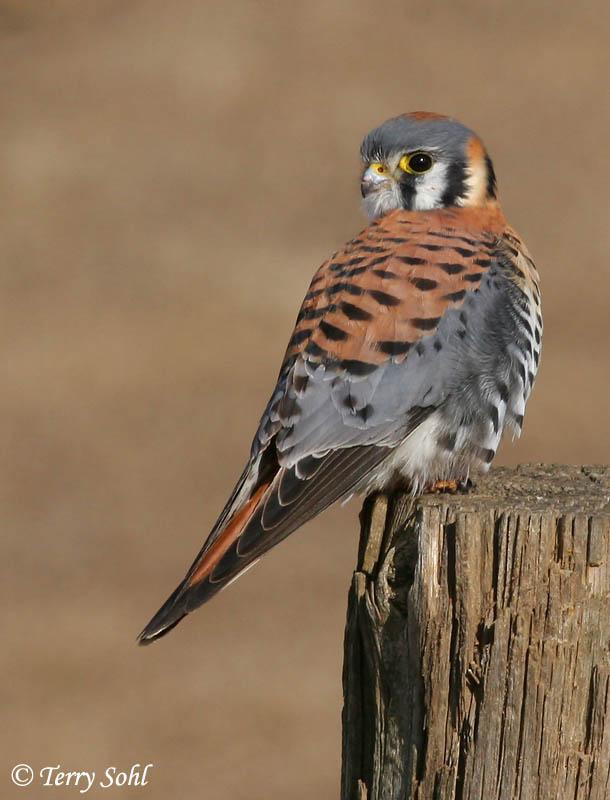The image features a small sparrow-like bird perched atop a weathered, sawed-off tree trunk, which appears old and dried. The bird has a gray head and chest, complemented by orange-brown feathers with black spots adorning its back. Its tail is dark brown with an orange streak. The bird's body is facing away, but its head is swiveled around, showcasing a black eye with a yellow iris that meets the camera's gaze. Beneath its eye, there's a distinctive white and black stripe, and its small beak is also white. Adding to the image's rustic charm is a brown background. In the lower left-hand corner, the text "Terry Sohl" is displayed in white letters against the brown backdrop.